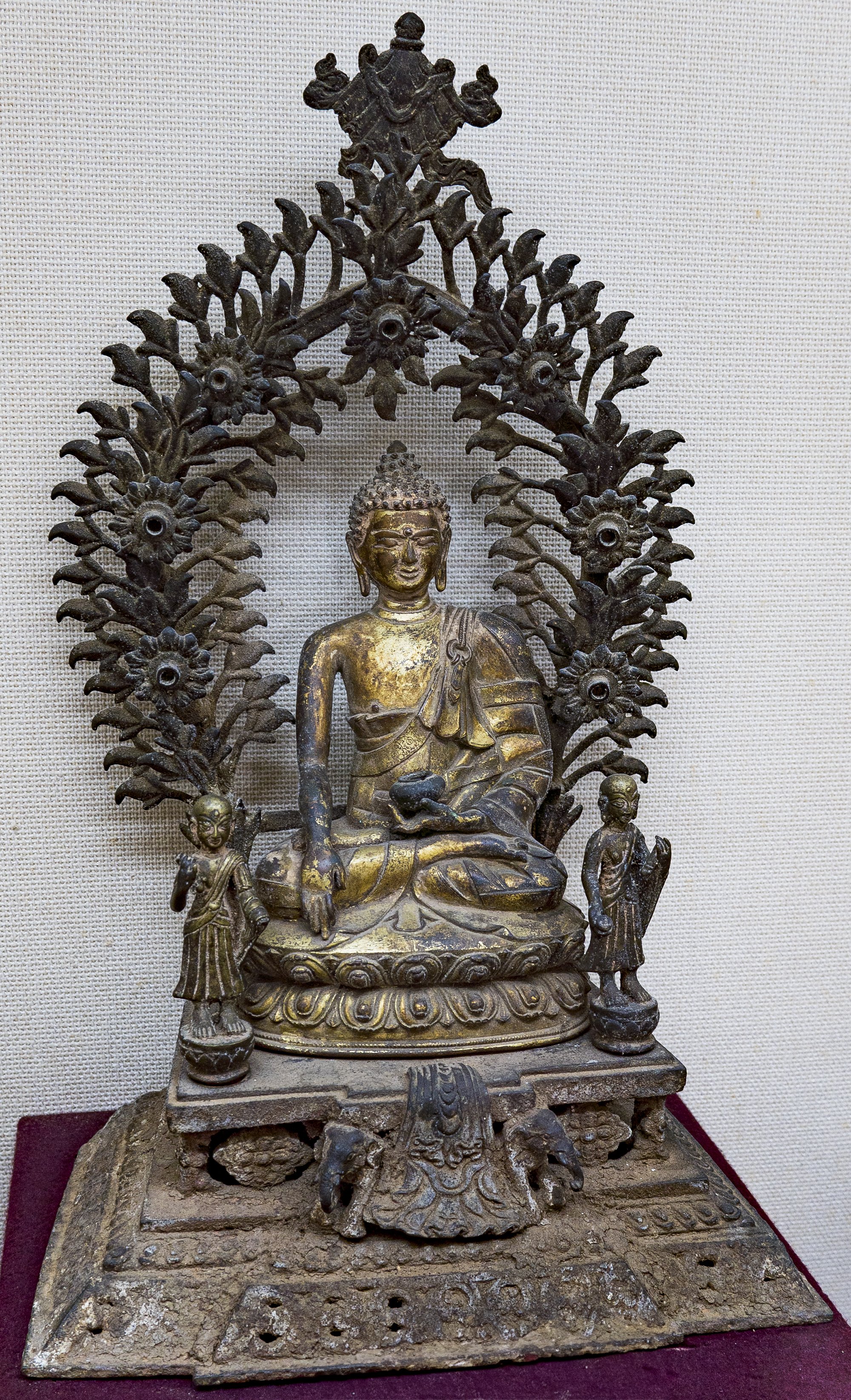This color photograph, captured in a portrait orientation, presents a detailed depiction of a bronze statue of Buddha situated on a table against a muted wall. The main focal point is a serene Buddha figure, centrally positioned and seated cross-legged. The Buddha features a pointed headgear and holds a black bowl in his left arm that rests over his lap, while his right arm is peacefully placed on his knee. Behind the Buddha is an elaborate wreath design with vines, crafted from bronze, that frames the serene visage and extends upwards into a decorative top. Flanking the central figure on each corner of the platform are two significantly smaller statuettes, identified as Shakyamuni, Sariputra, and Maudgalyayana. These details are set against a simple background, emphasizing the statue's intricate craftsmanship and tranquil aura.